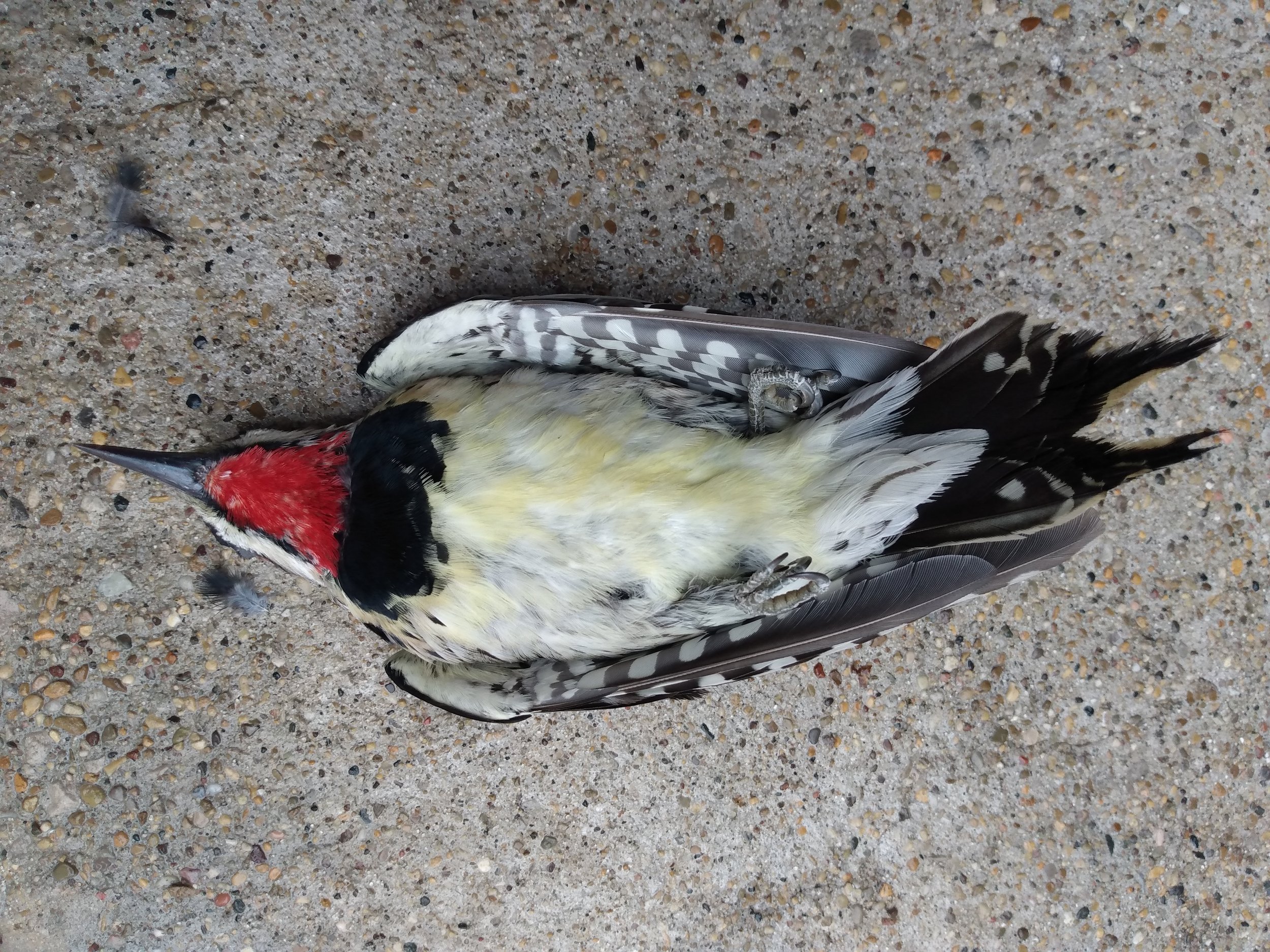This photograph captures a deceased bird lying on its back on a ground surface composed of various types of stones and speckled with colors like white, brown, black, and gray. The sharp beak of the bird is prominently visible, transitioning from a red fur-like texture beneath its mouth to black, with patches of red and a touch of yellow. The bird's body predominantly showcases a white underbelly with a slight yellowish hue. Its black and white wings display a distinctive striped or checkerboard pattern, with the white part where the wings meet the body. It has black, pointed tail feathers. The overall texture of the feathers varies; some parts appear smooth while others show a more pronounced furry texture.